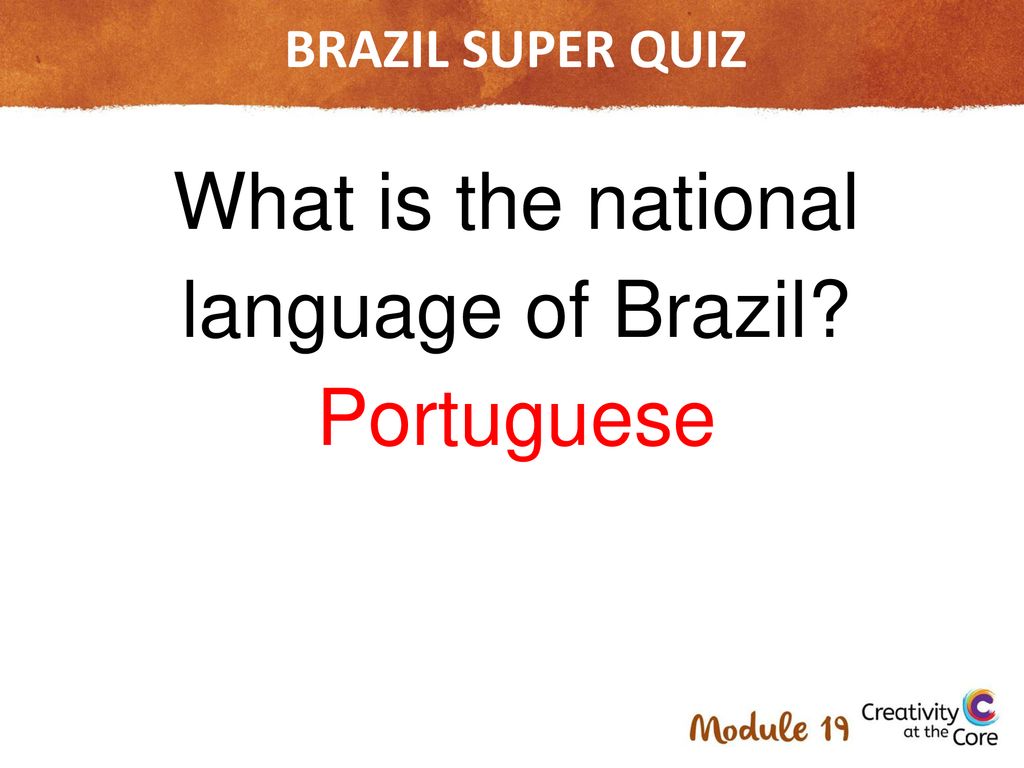The image depicts a language learning application interface. At the top, within a jagged, torn-paper-like rectangle colored in shades of brownish orange and gold, the text "BRAZIL SUPER QUIZ" is prominently displayed in bold, all-caps white letters. Below this rectangle, on a crisp white background, the question "What is the national language of Brazil?" is written in clear black text. The answer, "Portuguese," is highlighted in striking red letters directly underneath the question.

Towards the bottom right of the image, a gold inscription reads "Module 19," which appears more like a stylized logo or icon rather than simple text. Below the module indication, the phrase "Creativity at the Core" is written, accompanied by a uniquely designed letter "C." This "C" consists of multiple vibrant colors, starting from a purple core and radiating outward in gradients of yellow, orange, red, green, and finally transitioning into aqua blue.

Overall, the visual suggests this is a language quiz associated with the completion of Module 19, possibly focusing on Brazil, its national language, or language learning more broadly.